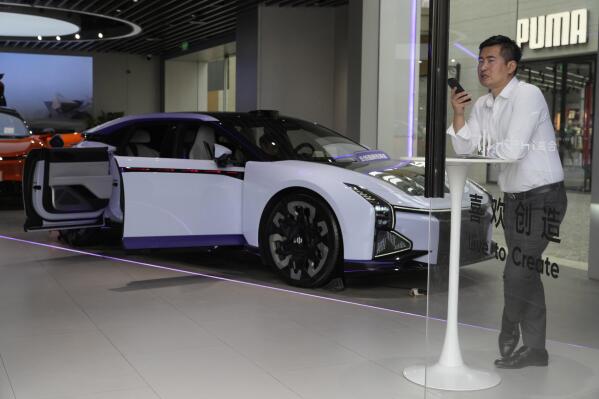The photo captures an indoor scene, seemingly set inside a sophisticated auto showroom or mall. The focal point is a sleek, lavender-colored sports car with distinctive purplish lines running across the rooftop and the bottom of the doors. Its doors are uniquely designed, with the front doors opening conventionally and the rear doors hinged at the back, creating an eye-catching display. Nearby, a partially visible red car adds to the luxurious ambiance. 

In the foreground, an Asian man is prominently featured, leaning against a small white cocktail table. He's engaged in a phone call on speaker, holding the black device casually. His attire consists of a white, long-sleeved, button-down shirt neatly tucked into black dress pants, complemented by black dress shoes and a matching belt. The man's polished look and relaxed posture suggest he might be a valet or an employee waiting for someone, adding a human element to the scene.

Through the glass window in the background, a Puma store across the street is clearly visible, giving context to the setting and hinting at an upscale environment. The floor beneath the car and man is gray, further emphasizing the modern, sleek atmosphere of the space.